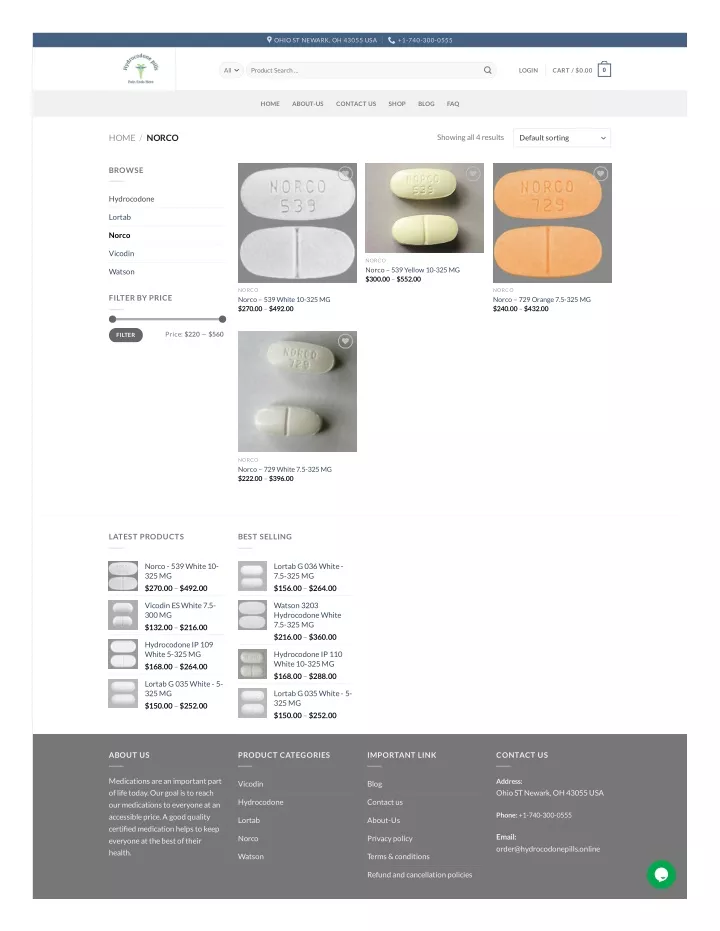This image showcases various medications, specifically different formulations of the pain reliever Norco. 

The image features several types of pills:
- A white pill with the imprint "Norco 539," which is priced between $270 to $492.
- A yellow pill labeled "Norco 539 Yellow 10-325mg," with a price range of $300 to $552.
- An orange pill identified as "Norco 729 7.5-325mg," costing between $240 to $432.
  
Additional pills are also listed in the image. The "About Us" section emphasizes the importance of medications in modern life. It outlines their mission to provide high-quality, certified medications at accessible prices to ensure everyone can maintain optimal health.